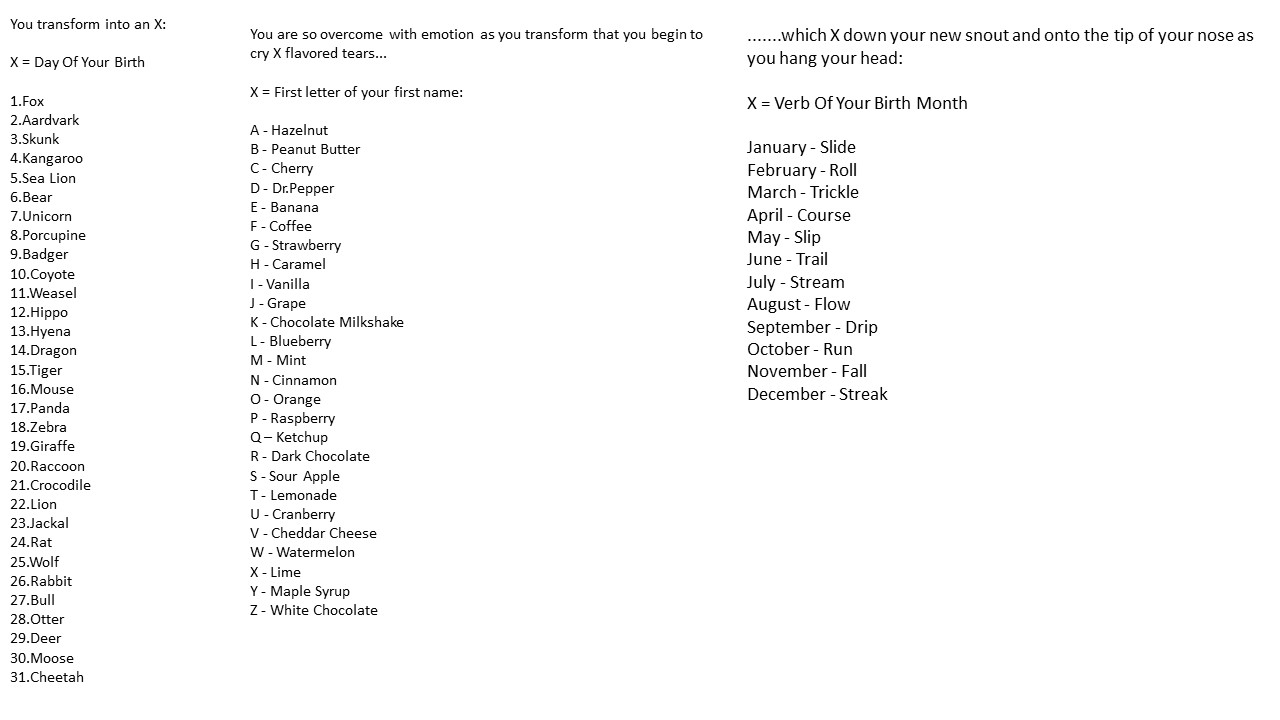This screenshot depicts a whimsical and imaginative chart titled "Your Transformation." The layout consists of three vertical columns against a stark white background, featuring black text. 

In the far-left column labeled "Day of Your Birth," the chart assigns an animal transformation based on the day you were born:
- 1: Fox
- 2: Aardvark
- 3: Skunk
- 4: Kangaroo
- 5: Sea Lion
- 6: Bear
- 7: Unicorn
- 8: Porcupine
- 9: Badger
- 10: Coyote
- 11: Weasel
- 12: Hippo
- 13: Hyena
- 14: Dragon
- 15: Tiger
- 16: Mouse
- 17: Panda
- 18: Zebra
- 19: Giraffe
- 20: Raccoon
- 21: Crocodile
- 22: Lion
- 23: Jackal
- 24: Rat
- 25: Wolf
- 26: Rabbit
- 27: Bull
- 28: Otter
- 29: Deer
- 30: Moose
- 31: Cheetah

The middle column, "First Letter of Your First Name," describes the flavor of your transformation tears:
- A: Hazelnut
- B: Peanut Butter
- C: Cherry
- D: Dr. Pepper
- E: Banana
- F: Coffee
- G: Strawberry
- H: Caramel
- I: Vanilla
- J: Grape
- K: Chocolate Milkshake
- L: Blueberry
- M: Mint
- N: Cinnamon
- O: Orange
- P: Raspberry
- Q: Ketchup
- R: Dark Chocolate
- S: Sour Apple
- T: Lemonade
- U: Cranberry
- V: Cheddar Cheese
- W: Watermelon
- X: Lime
- Y: Maple Syrup
- Z: White Chocolate

The final column, "Month of Your Birth," specifies a verb that describes the way your flavored tears move down your new snout:
- January: Slide
- February: Roll
- March: Trickle
- April: Course
- May: Slip
- June: Trail
- July: Stream
- August: Flow
- September: Drip
- October: Run
- November: Fall
- December: Streak

Thus, this intriguing chart creatively combines your birth information to imagine a surreal transformation scenario complete with emotional and sensory details.